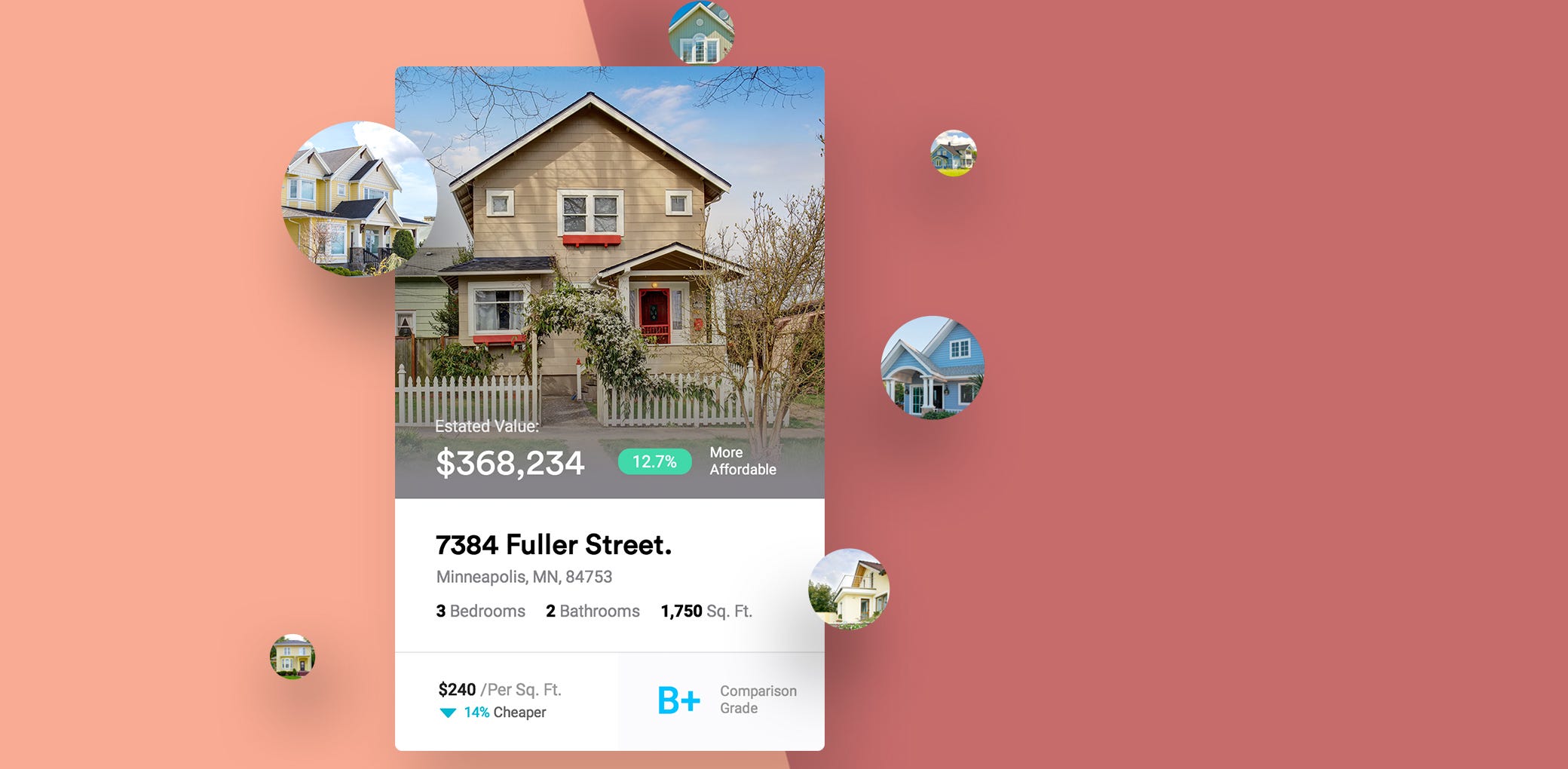The image depicts a vibrant website dedicated to evaluating home values. The background features a gradient transitioning from a coral orange to a darker pink, adorned with images of six different homes scattered across. At the center, where the orange fades into pink, there's an information sheet prominently displayed. This sheet showcases a dark beige house with white windows and red trim, listed with an estate value of $368,234. 

To the right of the house image, a teal box highlights "12.7% more affordable" in white letters. Additional property details are provided: the address is 7384 Fuller Street, Minneapolis, Minnesota, 84753, and the home includes three bedrooms, two bathrooms, covering a total of 1,750 square feet. The cost per square foot is stated as $240, which is noted to be 14% cheaper compared to similar properties. The comparison grade is marked as a B+, with both the "B+" grade and the "14% cheaper" notation presented in blue letters. All other details, except the estate value and affordability statement written in white, are rendered in black text.